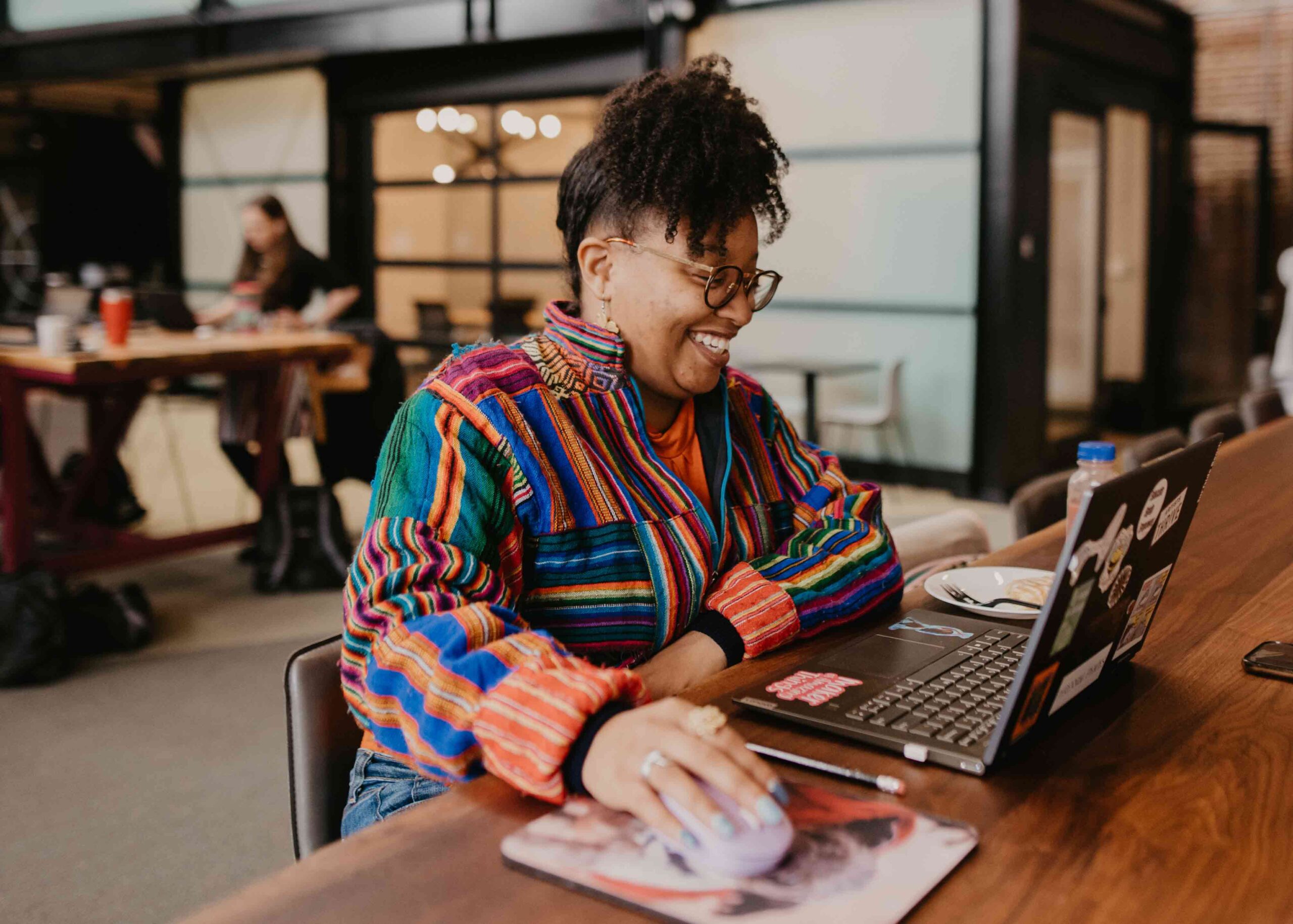In a vibrant, bustling cafe, an African-American woman with warm brown skin is engrossed in her work on a laptop adorned with numerous stickers. Her hair is stylishly piled atop her head, cascading over her forehead in a playful manner. She wears brown-framed glasses and a vividly colorful top that bursts with all the hues of the rainbow, paired with an orange shirt underneath a cozy zip-up hoodie. Her bright smile and occasional laughter light up the room as she uses a mouse to navigate her laptop. A plate with a fork and a bottle sit beside her on the wooden countertop, which is part of a long table surrounded by multiple chairs. In the background, other patrons, including a Caucasian woman, immerse themselves in their own activities, adding to the lively atmosphere of the cafe.